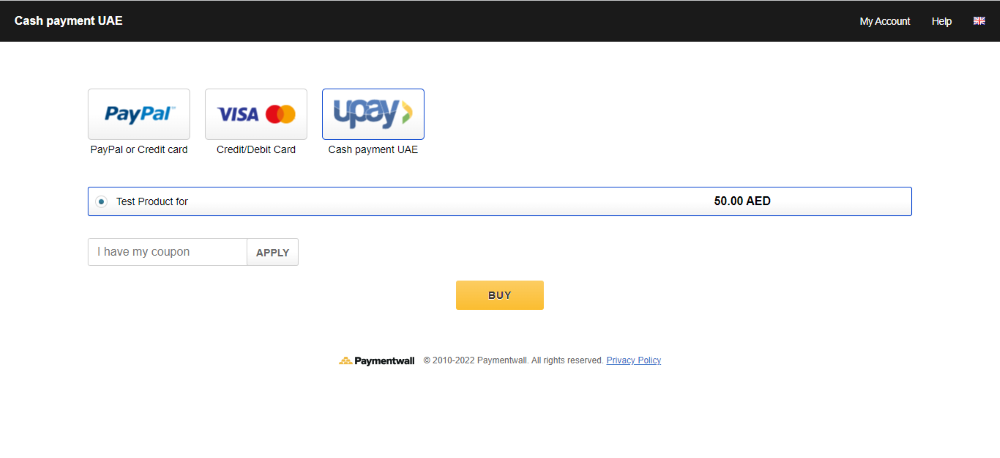The web page features a minimalist design with a white background. At the top left corner, a black ribbon houses the text "Cash Payment UAE" in white font. On the far right, the navigation options "My Account," "Help," and a country flag are displayed. Directly below this, there are three horizontally aligned buttons labeled "PayPal," "Visa," and "YouPay." Underneath each button, additional descriptions in black text read "PayPal or Credit Card," "Credit Debit Card," and "Cash Payment UAE," respectively.

A prominent white banner with a gray border spans the page below the buttons. Within this banner, a small blue dot precedes the black text "Test Product 4," and to the right, the price "50 AED" is displayed. Below this, a short white box contains the text "I have my coupon," accompanied by an "Apply" button to its right. An orange button centrally aligned and marked "Buy" in black text appears at the bottom, encouraging the user to proceed with the purchase.